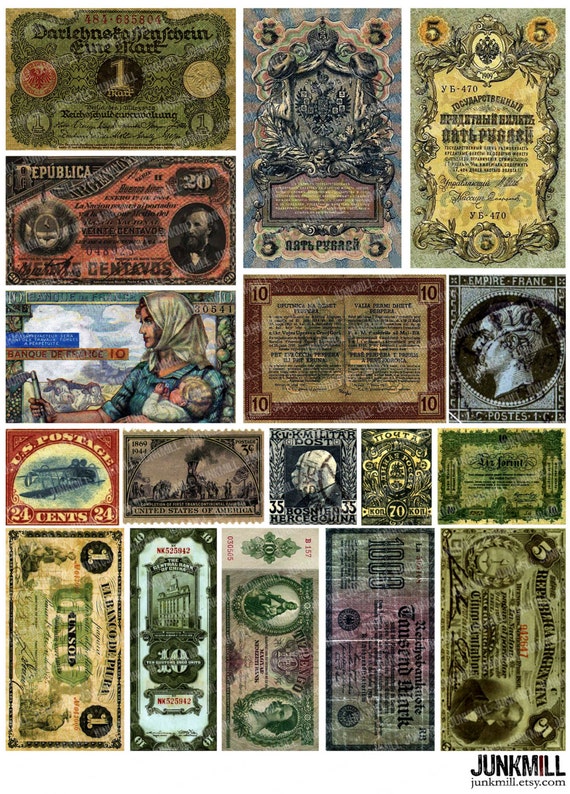The image displays an eclectic assortment of colorful paper money and postage stamps from various countries. Dominating the scene are numerous denominations of currency, ranging from $1, $5, $10, $20, and even some that are 35 and 70 units of an unspecified currency, in vibrant shades of green, dark green, yellow, blue, red, and pinkish-blue. Prominently featured are a $1 bill located at the top left, multiple $5 and $10 notes, and a $20 bill. Interspersed among the currencies are old and ornate postage stamps, including a French stamp, a 24-cent US stamp, several 3-cent US stamps, and various others. Each piece is richly colored and intricately designed, highlighting their historical and aesthetic significance. The bottom of the image bears a label reading "junkmill.etsy.com."